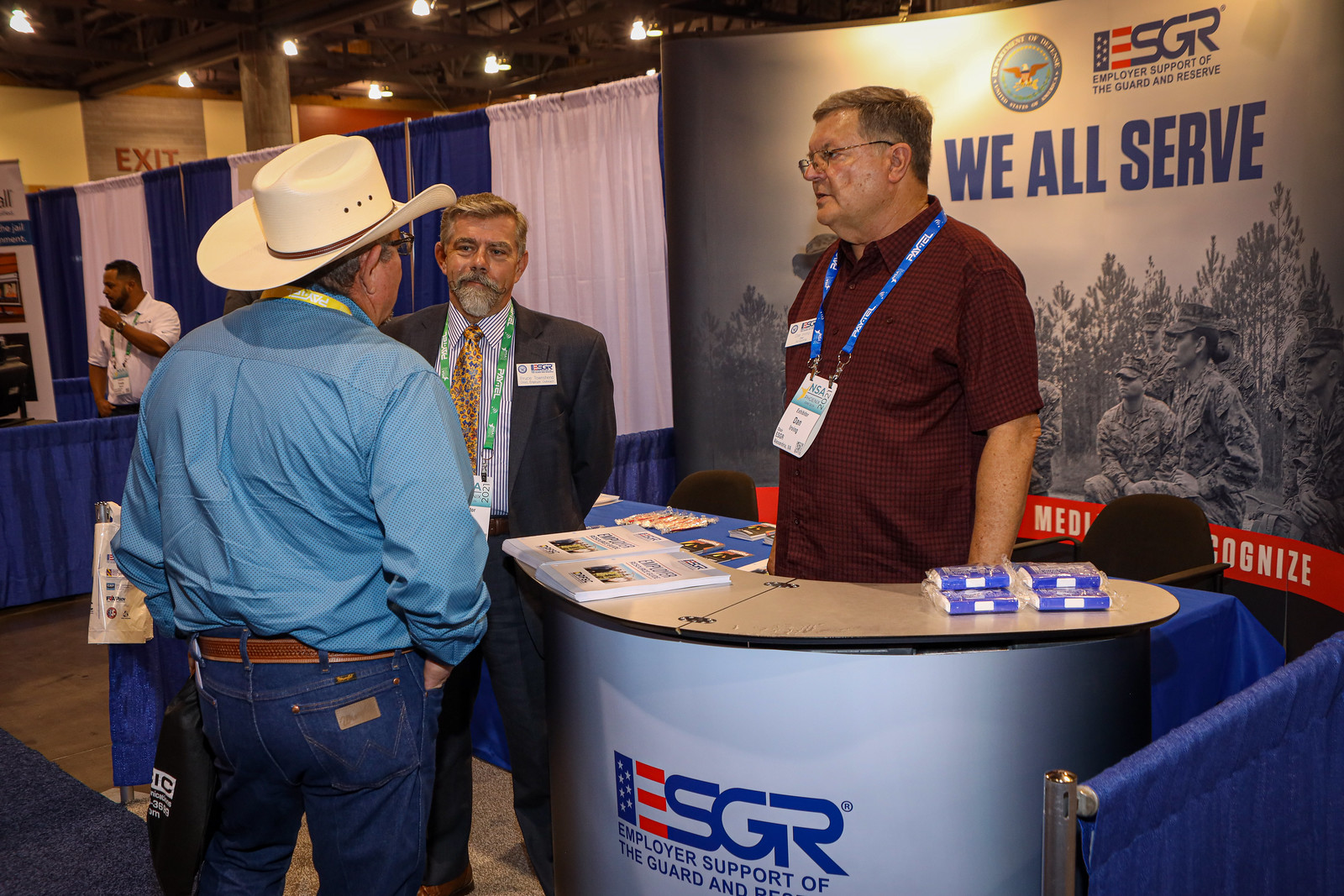In the horizontally aligned rectangular image, taken at an indoor conference or trade show, a man wearing a red button-down shirt with a small checked pattern and glasses stands behind a small, curved table with a brown top. The table, emblazoned with "ESGR" in red and blue letters and partially visible text "Employer Support of the Guard...," holds several items, including a book and stacks of papers. The man wears a blue lanyard and seems to be intently engaging with attendees. Directly in front of him, a man in a white cowboy hat, blue long-sleeved shirt, and blue jeans faces two others. One of these, positioned slightly to the left, sports a suit with a gold and black patterned tie and a name tag on his left chest, along with blondish-gray hair and a matching mustache and beard, and wears a green lanyard. The other, likely the red-shirted man mentioned earlier, contrasts sharply in his attire.

Behind them, a large wall displays the "ESGR, Employer Support of the Guard and Reserve. We All Serve" slogan, alongside a black and white image depicting trees and people in military uniforms. In the background, to the left, another table is set up with a man standing behind it, framed by blue and white curtains. The scene features various colors—blue, maroon, red, and more—set against the backdrop of hardwood flooring with scattered carpets, adding texture to the bustling conference ambiance.